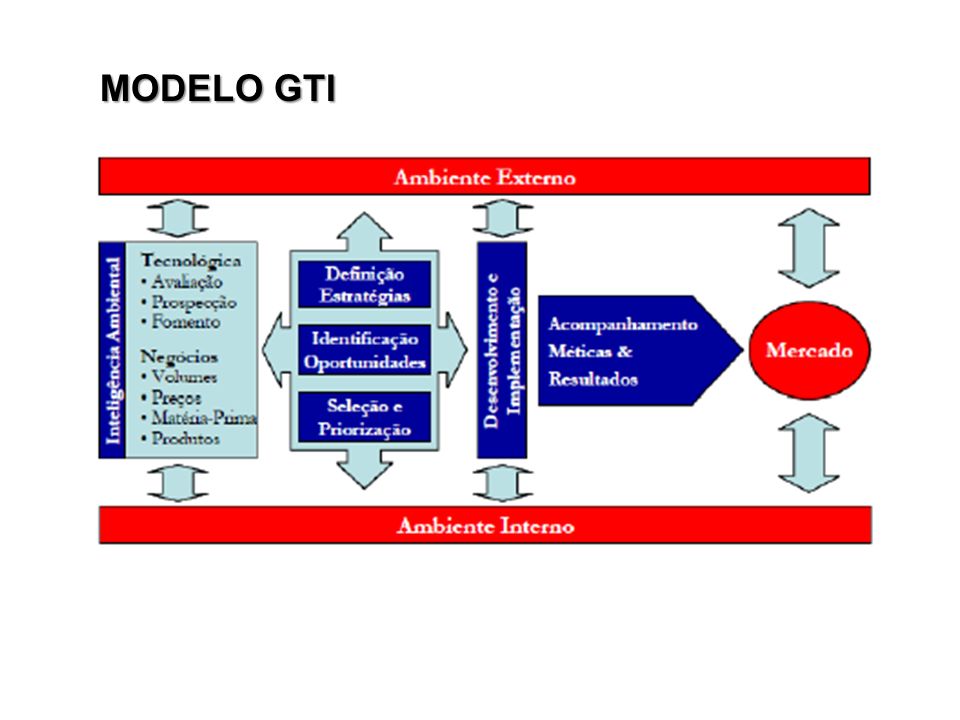This image is a detailed flowchart, likely in Spanish, labeled at the top with "Modelo GTI" in black letters. It features a thick red border at both the top and bottom. Inside the top red border, "Ambiente Externo" is written in white letters, and at the bottom, "Ambiente Interno" is similarly inscribed. The flowchart begins with a large blue rectangle, from which arrows extend both upwards and downwards on either side. Adjacent to this are blue blocks containing dark blue squares. As the chart progresses to the right, there is a thinner blue box followed by a large dark blue arrow pointing to the right. At the rightmost end, a prominent red circle contains the word "Mercado" in white letters, with arrows extending left and right on either side of the circle. The image includes various segments featuring light blue and dark blue boxes, filled with black and white text respectively, detailing components such as "Tecnología," "Negocios," "Definición Estratégica," "Implementación," and "Métricas y Resultados."